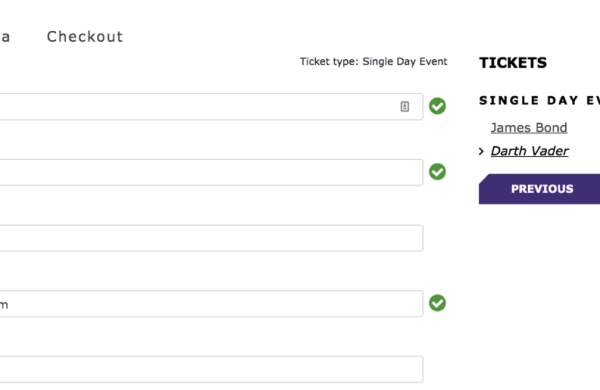An awkwardly cropped screenshot of an online checkout page for a single-day event. At the top, the word "Checkout" is prominently displayed. Below are elongated blank text fields indicating locations where user information is supposed to be entered; however, the entered details are cropped out of view. Green check marks next to each field imply that the information provided is accepted. The page shows a selection for "Ticket Type," labeled as a "Single Day Event," and peculiarly mentions fictional characters such as James Bond and Darth Vader, suggesting the event may involve these figures. The page also features a "Previous" button, allowing users to navigate back to earlier steps in the form. The background is predominantly white with black text, creating a stark contrast and a somewhat minimalist aesthetic. The overall context of the event remains unclear, with details about its nature being quite cryptic.